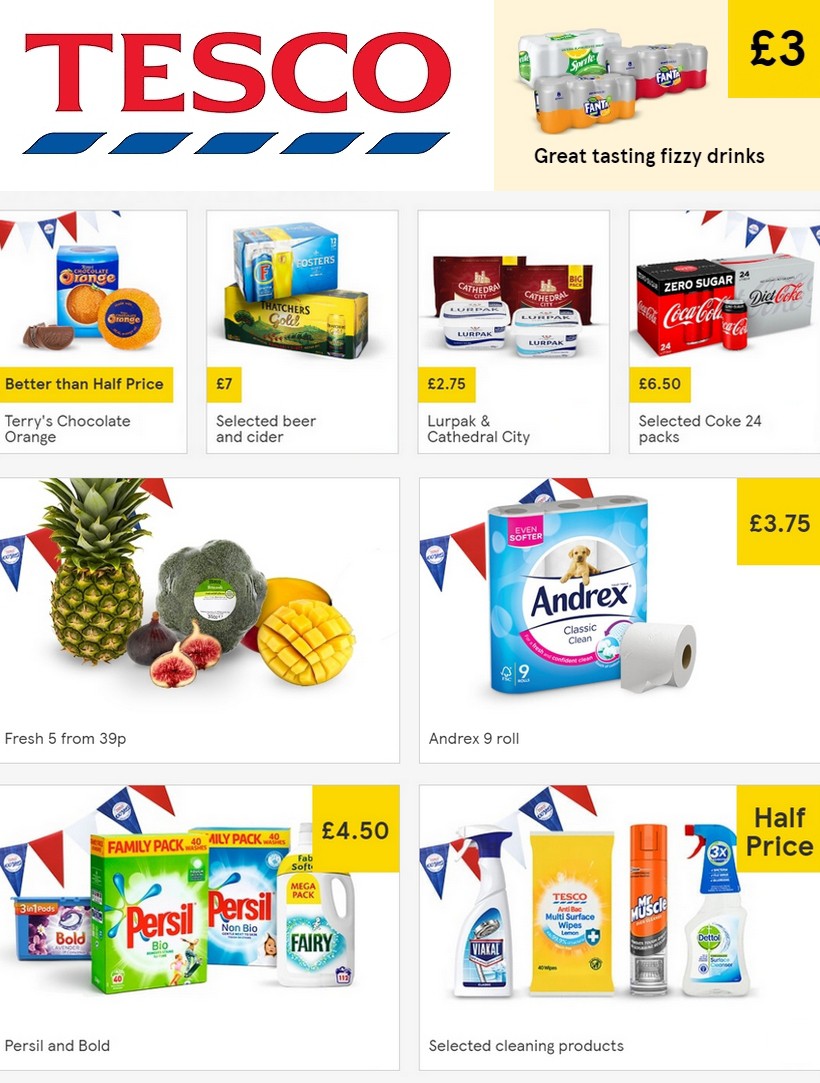This Tesco advertisement features the Tesco logo prominently in red at the top, with dotted blue lines below it. To the left, there are rolls of paper towels displayed. Moving to the right, there is a section showcasing great-tasting whiskey drinks priced at three pounds. Below, various items are listed, including orange juice, beer, and cider, indicating a mix of beverages available. The advertisement mentions Cathedral City, possibly indicating a local branch or product origin.

Coca-Cola and other soda options are prominently featured, situated next to images of pineapple and other fruits, emphasizing a variety of grocery items. On the right side of the advertisement, there are toilet paper rolls with some promotional copy on the packaging, demonstrating attention to household essentials. Additionally, there are cleaning supplies offered at half price, along with more cleaning products priced at $4.50. 

The advertisement uses yellow boxes for all price labels, making them easily noticeable. The overall layout appears to be a well-organized display of various product categories, from beverages and groceries to household essentials and cleaning supplies.